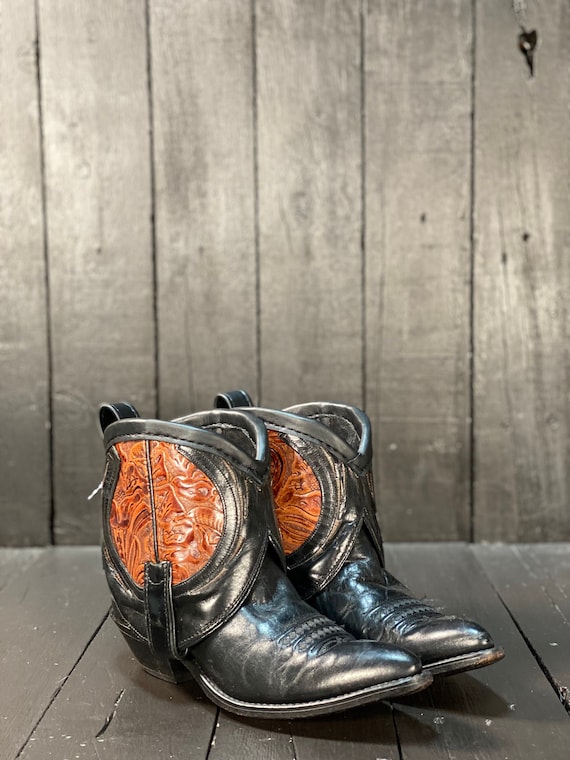This image showcases a pair of exceptionally stylized ladies' cowboy boots positioned on a weathered gray-washed wooden platform, against a matching background of the same material. The wood, comprised of worn and slightly scuffed slats, frames the boots, emphasizing their intricate design and craftsmanship. The boots are predominantly black, with a striking hand-tooled leatherwork that adorns the upper section, exhibiting a blend of orange-ish and brownish hues of tanned leather. Notably, the boots feature a sharp pointed toe and a moderate heel, tailored to make a fashion statement more than serve the functionality of traditional men's cowboy boots. Accentuating their stylish appeal, the boots include decorative silver trim, red design elements, and bootstraps on both the sides and back. Although they exhibit slight signs of wear, the boots retain their focus as the centerpiece of the photograph, distinguished by their unique aesthetics and detailing.